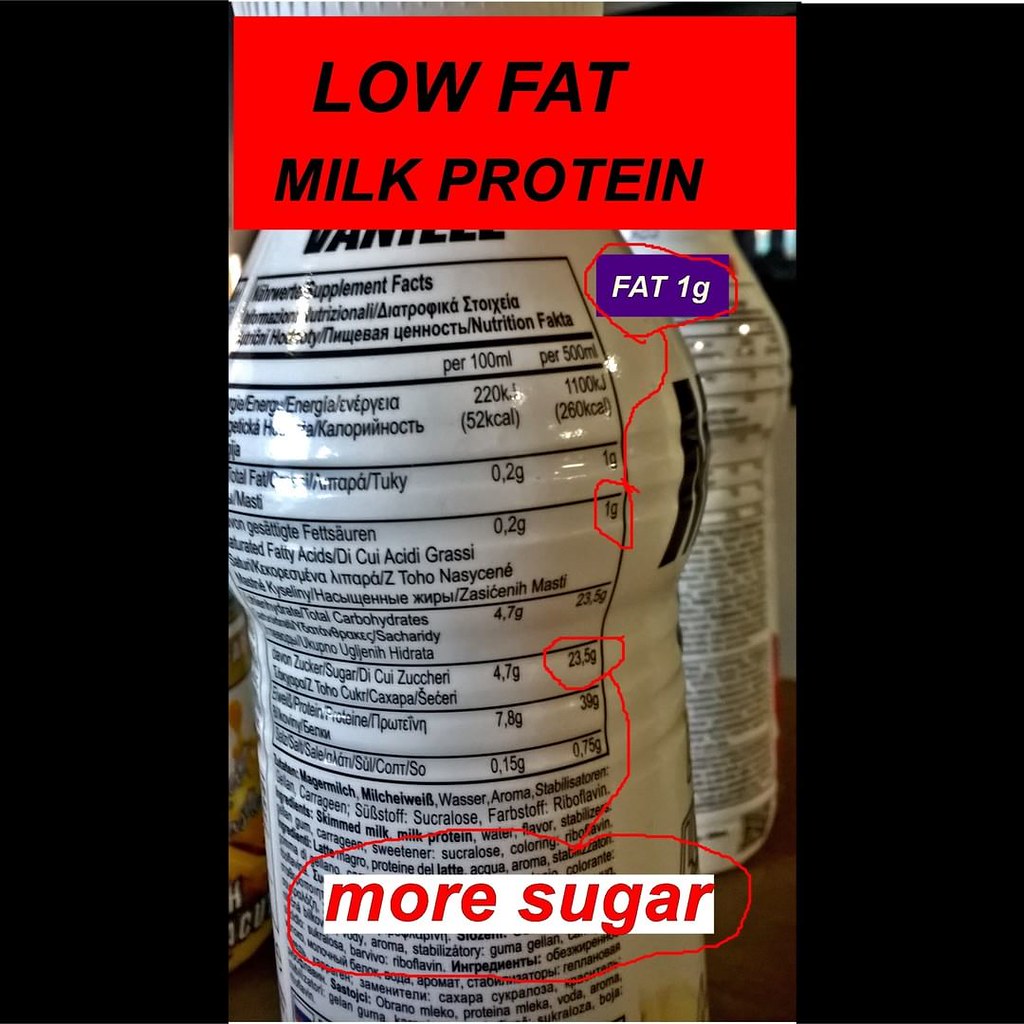The image is a color photograph, clearly marked up with digitized text to emphasize the fat and sugar content of a drink, albeit in a somewhat crude manner. It appears to have been edited on a mobile device, possibly using a basic photo editing app, rather than professional software, suggesting it was created to share an informal message with a friend rather than for advertising purposes.

At the top of the image, a red rectangle with black text stands out, declaring "Low Fat" on the first line and "Milk Protein" on the second. The image is presented in portrait orientation, but with black bars on either side, transforming the overall shape into a square.

The primary focus is on a bottle, specifically its back label, which is written in a foreign language, rendering most of the nutritional information unreadable to an English-speaking audience. However, certain details have been highlighted: "1 gram of fat" is circled in red, drawing attention to the low-fat content. Similarly, "23.5 grams of sugar" is also encircled in red, underscoring the high sugar content of the drink.

The makeshift and informal nature of the annotations, along with the clear emphasis on specific nutritional values, suggests that the image aims to inform or perhaps humorously point out a contrast between the drink's low-fat but high-sugar content.